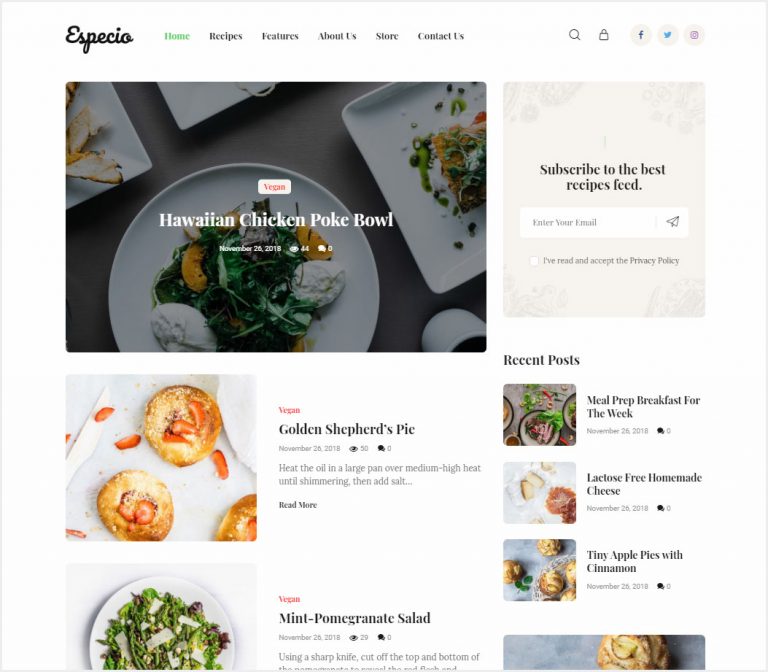The image depicts a web page dedicated to various categories, including Home, Recipes, Features, About Us, Store, and Contact Us. At the top right corner, there are icons for search (magnifying glass), cart or shopping list, and social media links for Facebook, Twitter, and Instagram. The webpage showcases several recipes with detailed information:

1. Hawaiian Chicken Poke Bowl - Posted on November 26, 2018, with 44 views and 0 comments.
2. Golden Shepherd's Pie - Posted on November 26, 2018, with 50 views.
3. Mint Pomegranate Salad - 29 views, 0 comments.
4. Meal Prep Breakfast for the Week - 0 comments.
5. Lactose-Free Homemade Cheese - 0 comments.
6. Tiny Apple Pie with Cinnamon - 0 comments. 

This detailed layout presents an inviting and user-friendly interface for visitors searching for meal inspirations and recipes.